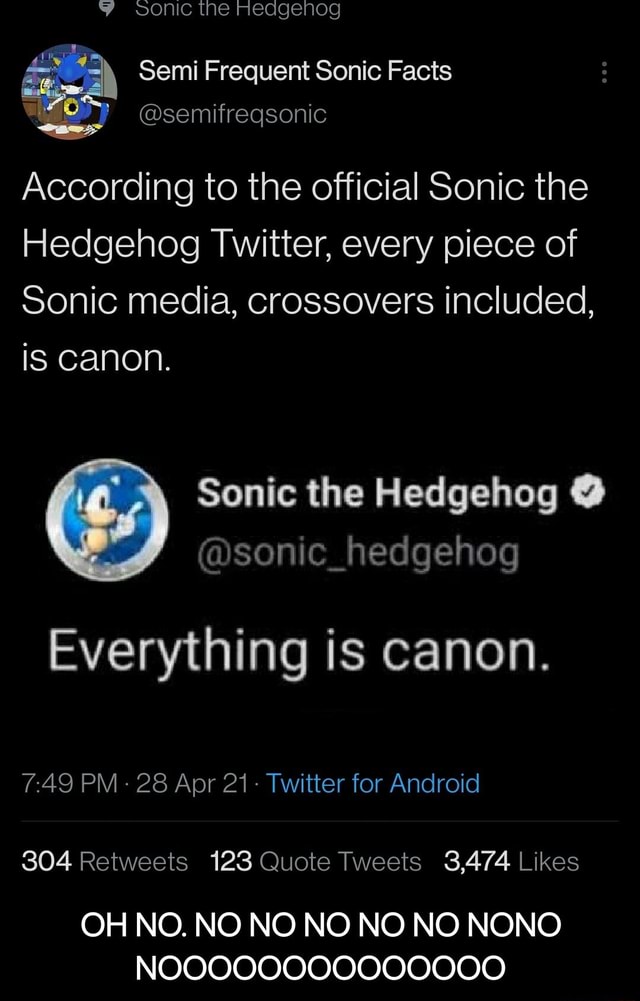This is a screenshot from the Instagram account SemiFrequentSonicFacts (@SemiFrequentSonicFacts). The post features an announcement from the official Sonic the Hedgehog Twitter account, which states: "According to the official Sonic the Hedgehog Twitter, every piece of Sonic media, crossovers included, is canon." Below this text, there is a snapshot of the referenced tweet from the Sonic the Hedgehog Twitter account (@Sonic_Hedgehog). The tweet displays in large, bold white text: "everything is canon." The time stamp on the post shows it was published at 7:49 AM on April 28th, 2021, via Twitter for Android. Engagement metrics reveal the tweet has amassed 304 retweets, 123 quote tweets, and 3,474 likes.